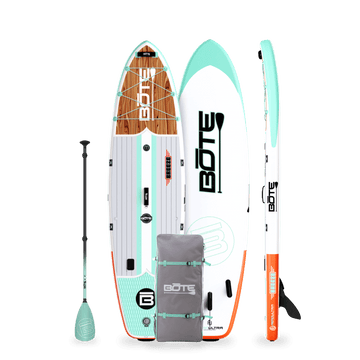The photograph features a detailed display of B-O-T-E branded water sports equipment against a stark white background. Central to the image are three surfboards standing upright, each showcasing unique color schemes. The surfboard on the left displays an intricate design with a wooden top portion, gray planking in the middle, accentuated with white and aqua stripes, and a blue bottom. The middle surfboard is primarily white with a blue top and has the B-O-T-E logo emblazoned in bold black letters. On the right, the surfboard is viewed from the side, revealing a gradient of blue at the top, transitioning to white, and finishing with orange at the bottom, complete with a black fin for improved hydrodynamics.

Accompanying the surfboards is a light aqua paddle which features a black handle, positioned to the left of the boards. In front of these, there is a purple backpack-like bag with aqua straps and the B-O-T-E logo prominently displayed in white. The meticulous color coordination extends across all items, with a cohesive palette of light aqua, white, gray, black, and orange, underscoring the brand’s distinct aesthetic.